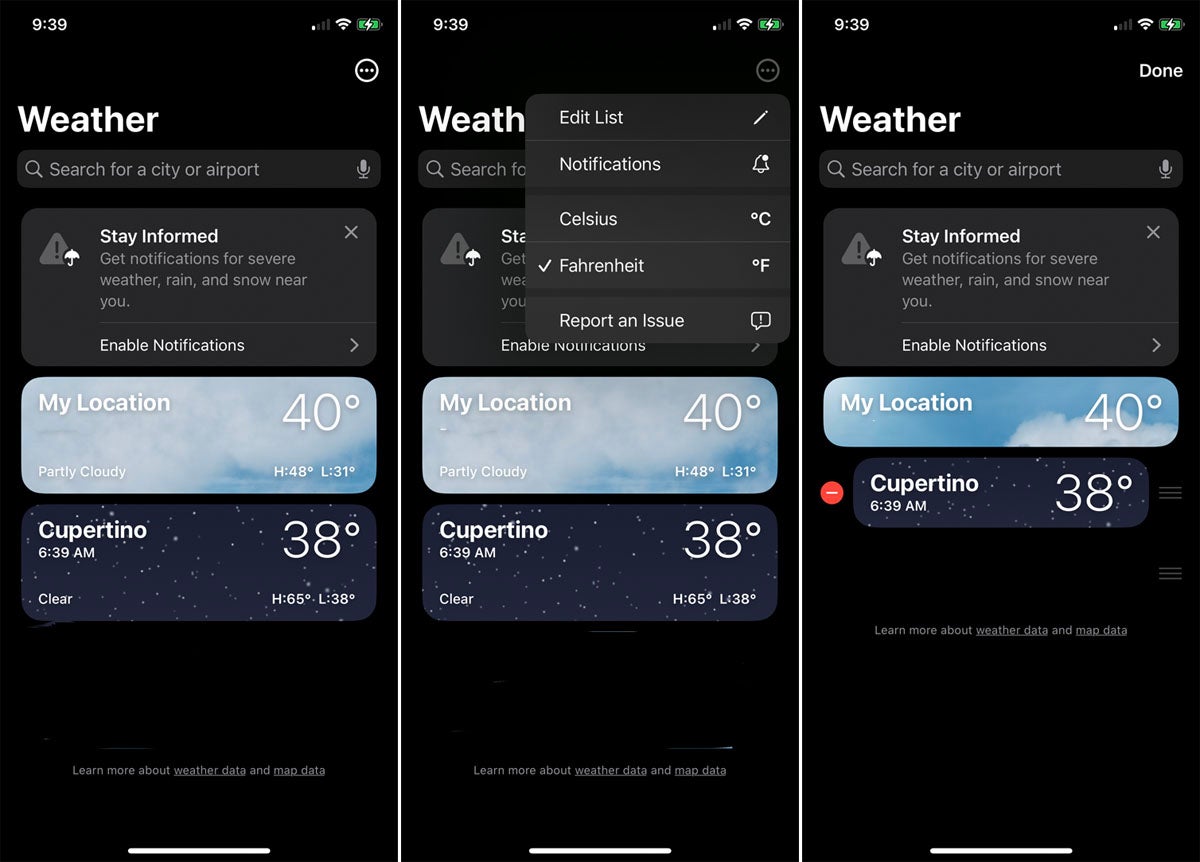The image displays three smartphone screenshots showcasing weather information. Each screenshot is taken at 9:39 AM and displays identical battery and Wi-Fi icons. Here’s a detailed breakdown from left to right:

1. **Left Screenshot**: 
   - Displays a weather application with a search box labeled "Search for a city or airport."
   - Below the search box, there’s a prompt to "Stay informed: Get notifications for severe weather, rain, and snow near you" with an option to enable notifications.
   - The weather is set to "My Location" with a current temperature of 40°F. The high for the day is 48°F, and the low is 31°F.
   - Cupertino's local time is shown as 6:39 AM with a clear status, and the high and low temperatures as 65°F and 38°F, respectively.

2. **Middle Screenshot**: 
   - Identical to the left screenshot in terms of weather display and location details.
   - Contains an additional pop-up box with options to "Edit List Notifications, Isabelle Celsius" with Celsius symbol, "Fahrenheit" with Fahrenheit symbol (checked), and "Report Issues."

3. **Right Screenshot**: 
   - Similar structure with the search box and notification prompt.
   - Shows the current location weather at 40°F without the high and low daily temperatures.
   - Cupertino's time remains at 6:39 AM but lacks details on weather conditions and the high/low temperatures. Instead, a red circle with a negative symbol is visible likely indicating an error or alert.

All three screenshots emphasize the weather application’s consistency across different scenarios while highlighting minor differences in weather data and interface features.